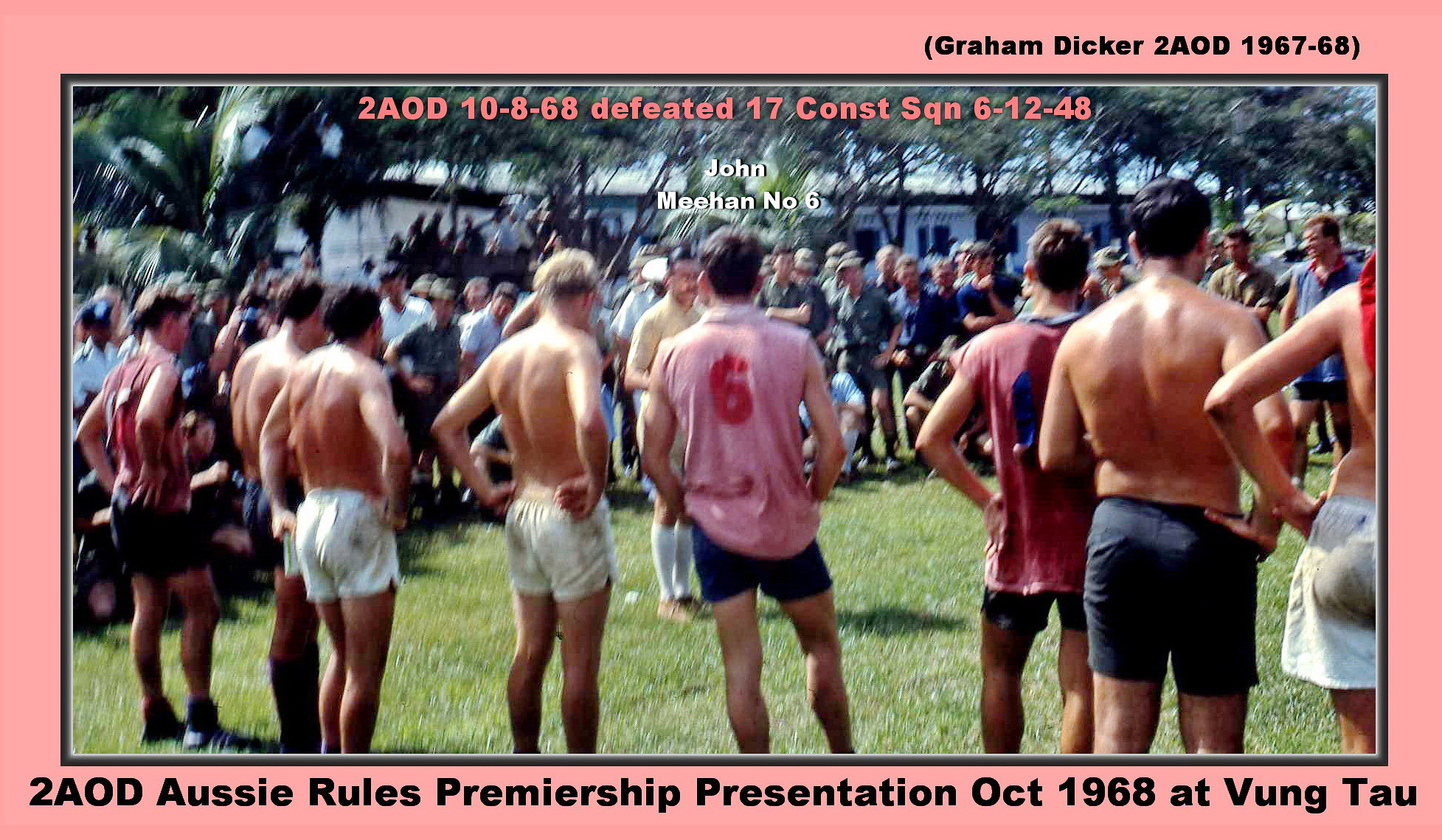This is a full-color landscape photograph from October 1968, capturing a scene from an Aussie Rules Premiership presentation in Vung Tau, Vietnam. The daytime image shows a group of approximately eight men, most of whom are shirtless while a few wear red shirts. They all don black or white shorts. Notably, one of the men in the center is wearing the number six, identified as John Meehan. The men are standing on a grassy field, with a blurred background featuring around 20-30 more fully clothed people, a building, and some trees. The photograph's narrow black border is encased in a wider pink border. Text within this pink border in the upper right reads, "Graham Dicker, 2AOD 1967-1968," and at the bottom, it states, "2AOD Aussie Rules Premiership Presentation, October 1968 at Vung Tau." Additionally, within the photograph, pink text reads, "2AOD 10-8-68 defeated 17 Const SQN 6-12-48," emphasizing the event's significance.